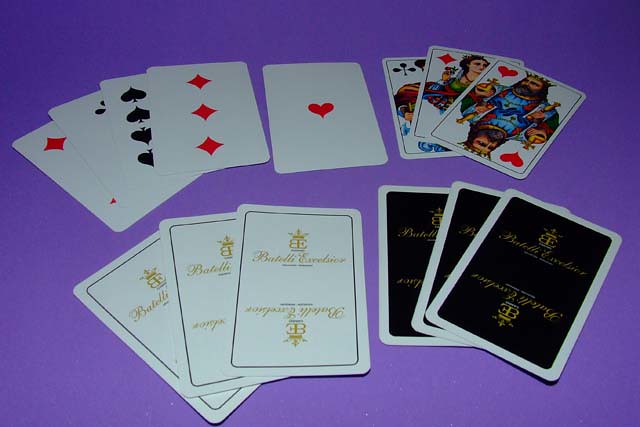In this vibrant photograph of playing cards, the layout is artistically arranged on a purplish surface, creating a striking contrast. In the top row, four cards are elegantly splayed out, featuring a diamond, a spade, another diamond, and a heart suit, adorned with detailed illustrations of kings and queens in rich blues, reds, and golds on a white background. Off to the side, three additional cards are displayed: a clover, a diamond, and a heart. On the bottom row, the cards are facing in the opposite direction, organized into two groups of three. The first group consists of white cards with gold lettering, while the second group comprises black cards with gold lettering, each adorned with delicate writing and a small symbol, differing only in color. The carefully chosen background elevates the visual allure of the entire arrangement, highlighting the intricate details and vivid hues of the playing cards.